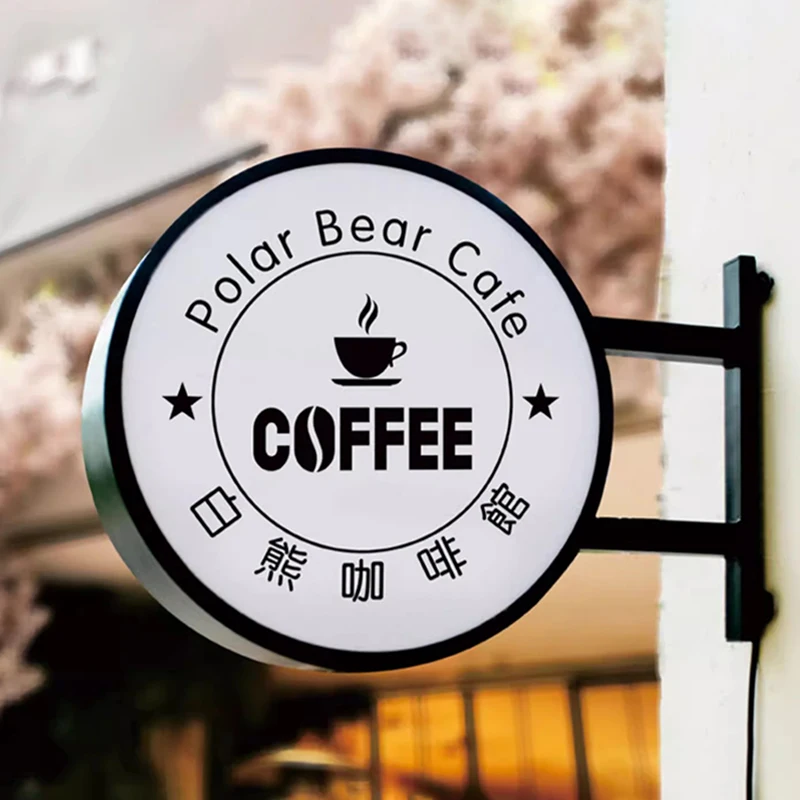The image shows a signboard for the Polar Bear Cafe, prominently featuring a white circular design with a black border. Centered within the circle, the upper section displays the text "Polar Bear Cafe" along with two black stars on either side of the word "coffee," which has a coffee bean incorporated into the letter 'O.' Below this, there are intricate Japanese or Chinese characters. The sign is affixed to a white wall and supported by a black pole. In the blurred background, there are hints of buildings and trees with pink flowers, suggesting a picturesque setting.